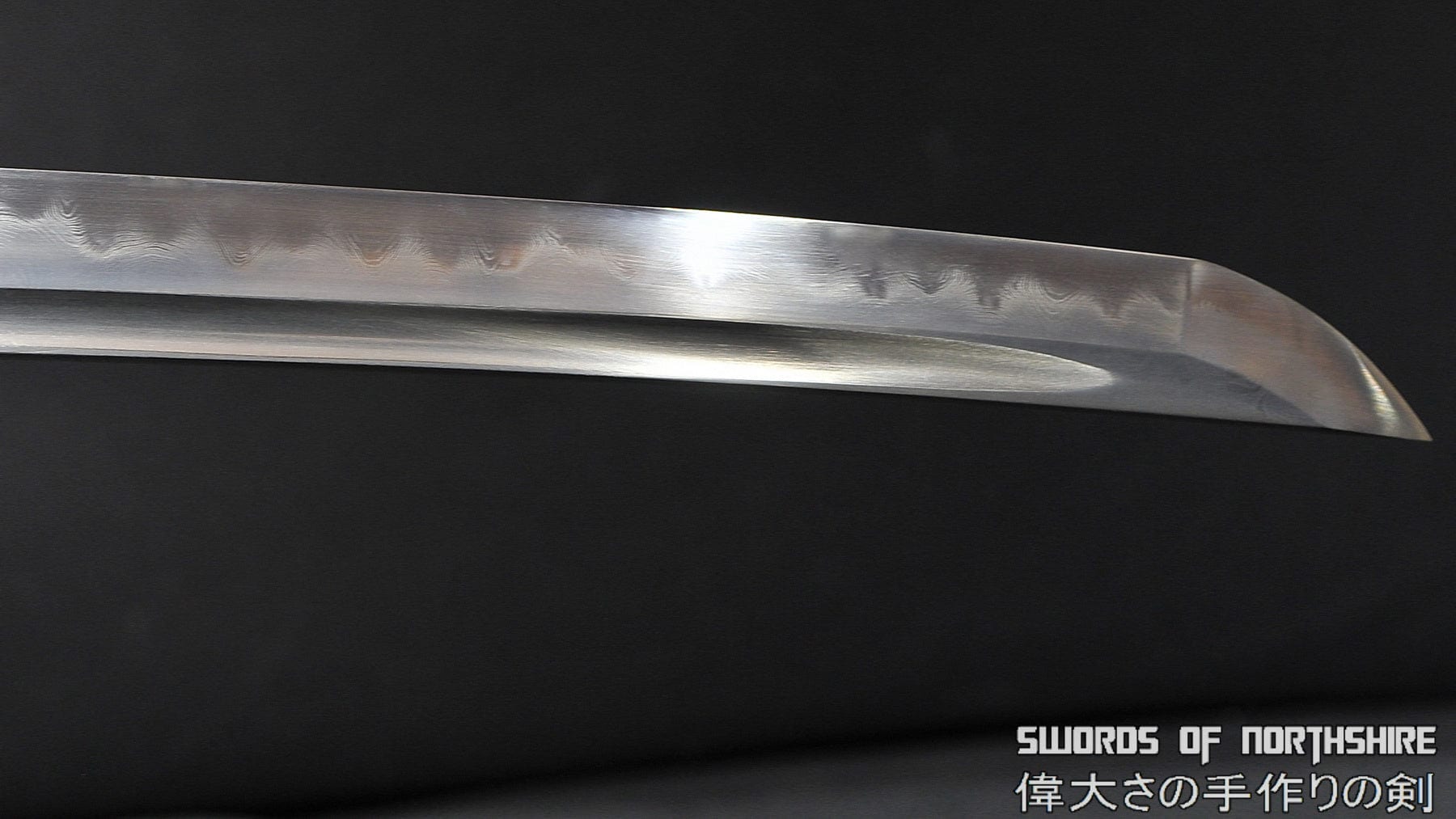Against a black background, this photograph prominently features an upside-down silver sword blade. The focus is on the blade's pointy tip and its smooth surface, showcasing the detailed wavy, water-like pattern resulting from its sharpening process. The sword, reminiscent of a Japanese design, has its cutting edge along the upper side, curving down to a distinctly sharp tip. Below the blade, in bold, white, capital letters, is the text "SWORDS OF NORTHSHIRE," which stands out against the dark background. Beneath this, there is additional text in Chinese characters, also in bold, reinforcing the emphasis on the sword's craftsmanship and origin. The composition uses the contrasting dark gray and black tones to make the shiny metallic blade glisten and pop within the image.